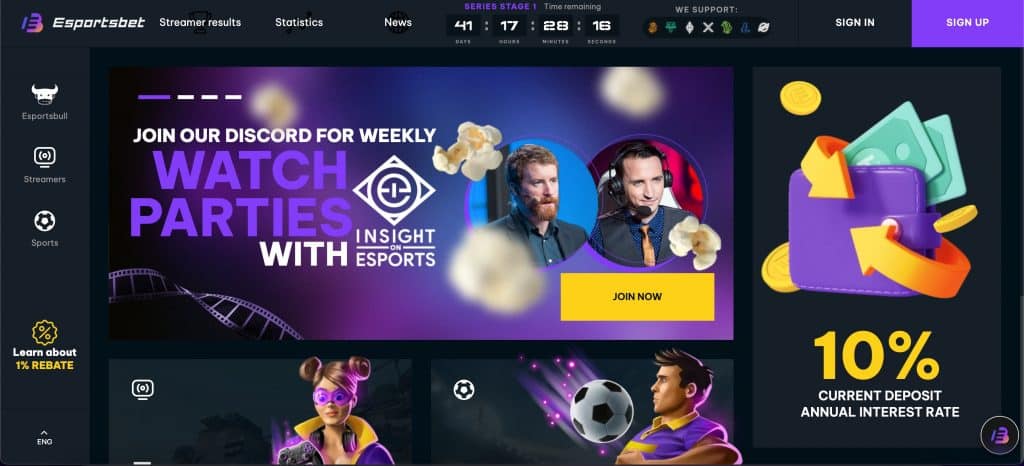In the image, the background is dark, creating a dramatic contrast for the white text. Starting from the top left, the page name "eSportsBets" is prominently displayed with a purple "e" symbol to the right of it. Directly below, there are navigation tabs labeled Streamer Results, Statistics, and News.

A timer positioned beneath these tabs indicates 41 days, 17 hours, 28 minutes, and 16 seconds remaining for Series Stage 1. The top right corner features "Sign In" and "Sign Up" options, with the "Sign Up" button highlighted in purple.

On the left side of the page, a sidebar menu includes links to eSportsPool, Streamers, and Sports. Towards the bottom of this sidebar, a yellow banner reads "Learn about 1% rebate."

Dominating the center of the page is a call to action: "Join our Discord for weekly watch parties with insight on eSports." The phrase "watch parties" is written in purple, while the rest of the text appears in black on a dark purple background. Near this, two Discord user icons are displayed on the right side. Below the call to action, a yellow button labeled "Join Now" stands out amid flying white popcorn kernels.

At the bottom left, an image depicts a female wearing purple and yellow, holding a black joystick, hinting at gaming. Next to her, a soccer player in action is seen placing a black-and-white soccer ball against their chest. On the bottom right, a banner highlights a 10% current deposit offer with a purple wallet, green paper bills, and a yellow arrow. The text "10% current deposit are not interested" is written in white.

Overall, the image is a rich tapestry of vibrant colors and engaging elements designed to draw in eSports enthusiasts.